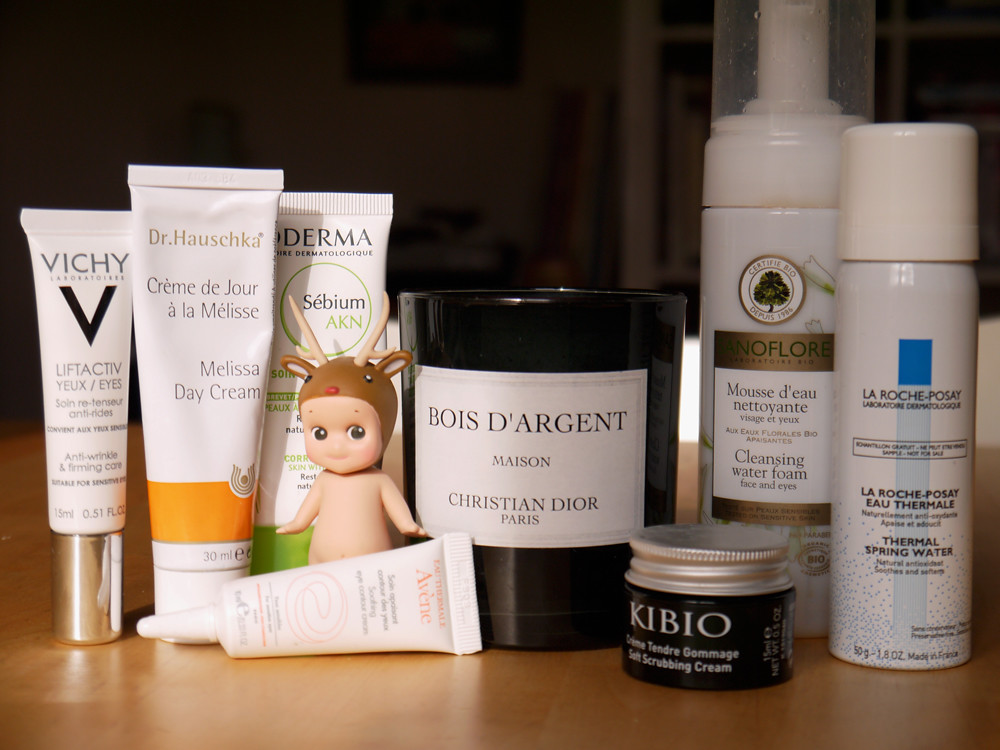In the photograph, a light brown wooden table is beautifully arranged with an array of skincare products and a small figurine. The scene is bathed in focused lighting, which highlights the items on the table while the background remains dimly lit, revealing just the outlines of what appears to be a room with large cupboard storage and possibly a television mounted on the wall.

From left to right, the products are meticulously placed:

1. **Vichy Liftactiv Eye Cream**: A white tube with gold trim, prominently marked in both French and English as an anti-wrinkle and firming eye care cream. It stands upright on its gold lid.
2. **Dr. Hauschka Melissa Day Cream**: A slender white bottle with an orange trim and logo, labeled in both French and English. The 30-milliliter bottle is standing on its white cap.
3. **Unidentified Derma Product**: Partially obscured by a quirky figurine of a small, naked character with a reindeer headpiece, this product has a green lid and the letters "CBMAKN" visible in the name. It stands on its lid, adding a touch of mystery to the collection.
4. **Eau Thermale Avène Cream**: While the specifics of this product remain unclear, its subtle presence adds to the diversity of the collection.
5. **Christian Dior Bois d'Argent Candle**: A luxe black candle with a crisp white label, marked with 'Maison Christian Dior Paris,' offering a sense of opulence and soothing fragrance.
6. **Certifié Bio Cleansing Foam**: This eco-friendly product boasts a spray pump mechanism, marked as 'de Plus Mousse de Nettoyant,' ideal for thorough cleansing.
7. **La Roche-Posay Thermal Spring Water**: A facial spray known for its soothing properties, adding a touch of elegance and simplicity to the lineup.
8. **Kibio Soft Scrubbing Cream**: Positioned at the front, this black container with a tin lid ensures smooth and gentle exfoliation.

The little figurine with the reindeer head adds a delightful and whimsical touch to the otherwise sophisticated array of skincare essentials, harmonizing the practical with the playful.